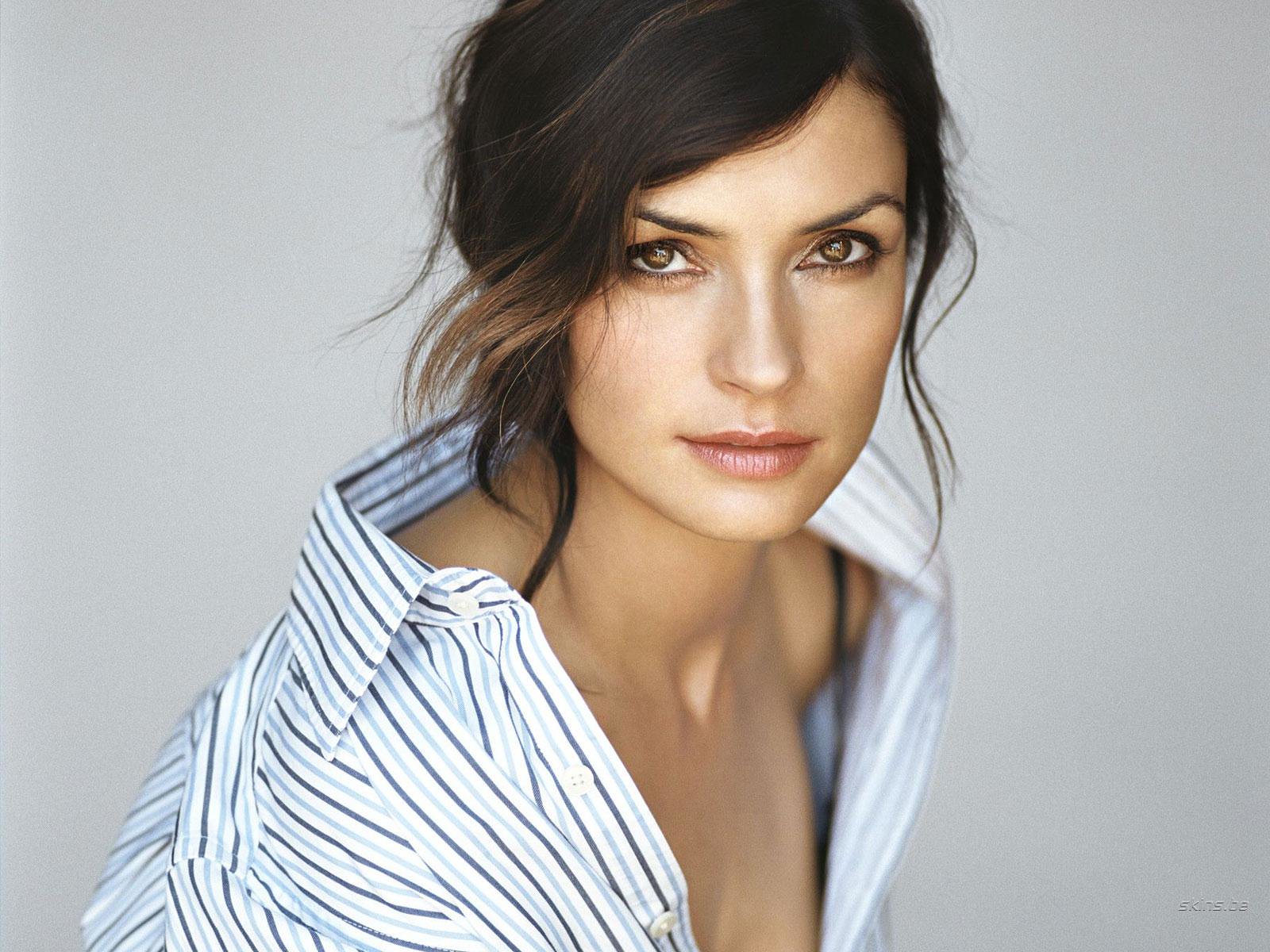This professionally taken portrait features a woman, likely Femke Jensen, positioned centrally against a gray background. She gazes directly at the camera, her body slightly angled in profile. Her dark brown, wavy hair is styled with a few strands delicately framing her face, while the rest is pulled back into a low, messy ponytail. She has striking amber-tinted brown eyes accentuated by dark eye makeup and paired with light lipstick.

The woman is dressed in a white, oversized button-up shirt adorned with light and dark blue vertical stripes. The shirt is casually draped over her shoulders, revealing a glimpse of her skin and a dark-colored strap, possibly from a tank top underneath. The background's muted tones are complemented by the simplicity of her outfit and the overall aesthetic of the photograph. In the bottom right corner, there is a nearly transparent but slightly visible logo that reads "Skins.be," hinting at the image's professional and studio setting.